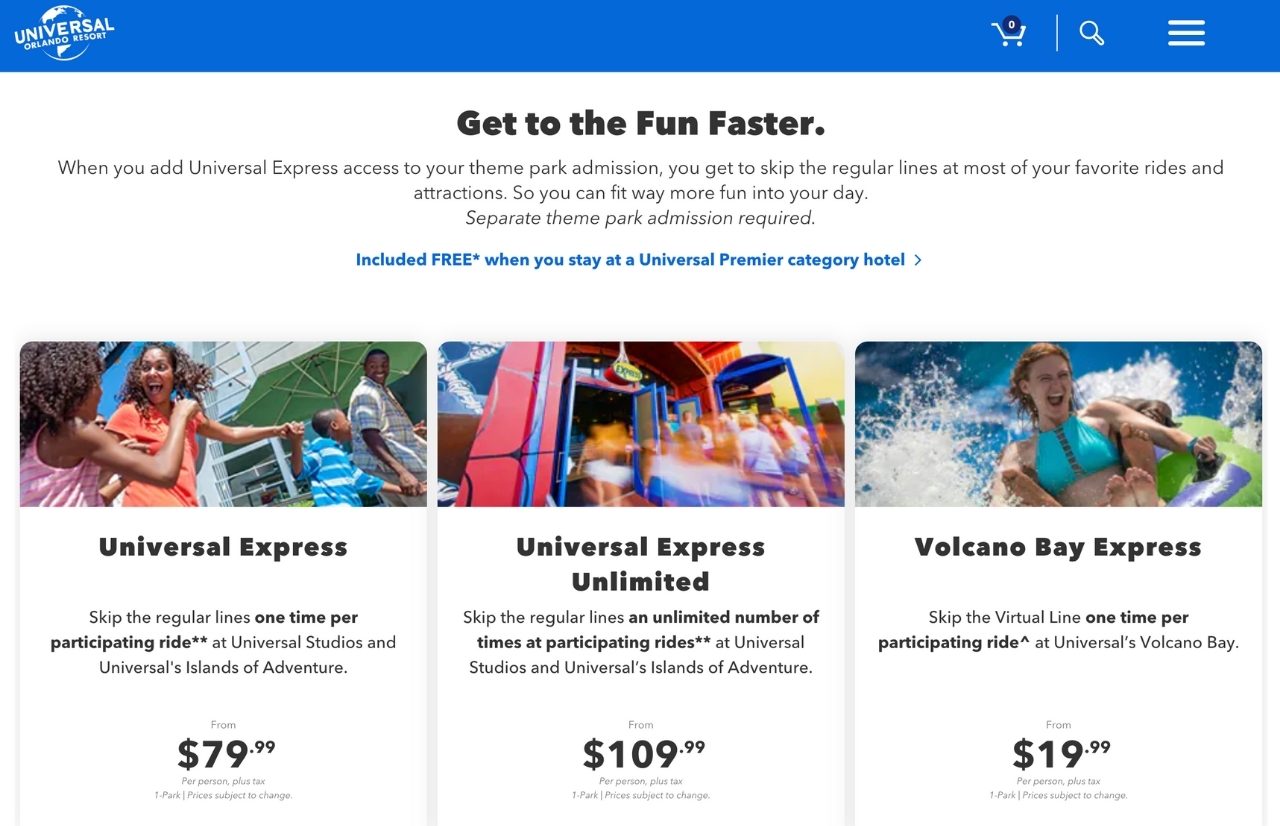The desktop version of the Universal Orlando Resort website features a vibrant, bright blue header at the top. The left side of the header prominently displays the Universal Orlando Resort logo, which consists of a globe with the company name. On the right side of the header, there is a shopping cart icon with items in the cart, a search icon, and a menu indicated by three white horizontal lines for additional navigation options.

Below the header, the main content of the webpage promotes the Universal Express passes with the heading "Get to the fun faster. Learn about the Universal Express." The page lists various options and prices for the passes: Universal Express starting at $79.99, Universal Express Unlimited providing unlimited usage for skipping regular lines at participating rides, and Volcano Bay Express for $19.99, which allows visitors to skip lines specifically at Universal's Volcano Bay water park. The prices mentioned are the starting rates, with a clickable option for more detailed information and additional pricing.